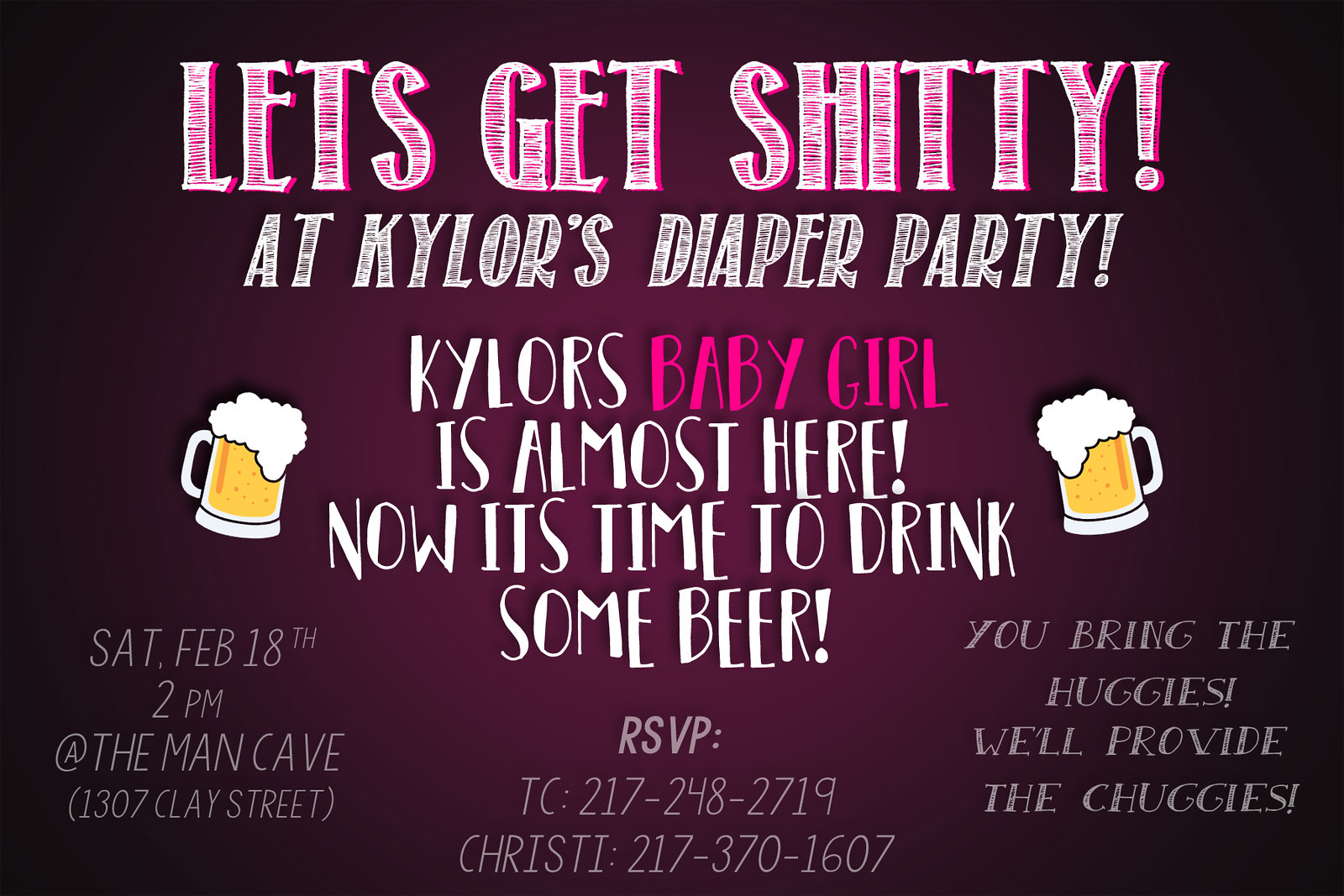The advertisement for Kylor's diaper party features a striking design with a predominant black background on the left and right sides, transitioning to an amber color in the middle. At the top, bold white letters with red brush strokes proclaim "Let's Get Shitty," followed by "At Kylor's Diaper Party" in white text with black lines through it. Below, it enthusiastically announces, “Kylor's Baby Girl is almost here. Now it's time to drink some beer.” On either side of this central text are decals of frothy coffee mugs. The bottom left corner provides event details: "Saturday, February 18th, 2 p.m., at The Man Cave, 1307 Clay Street." Centrally at the bottom, the RSVP contacts are listed: "TC, 217-248-2719" and "Christy, 217-370-1607." The bottom right corner declares, "You Bring the Huggies, We'll Provide the Chuggies." The image's clarity is bright and easy to read, effectively drawing attention to the festive details.